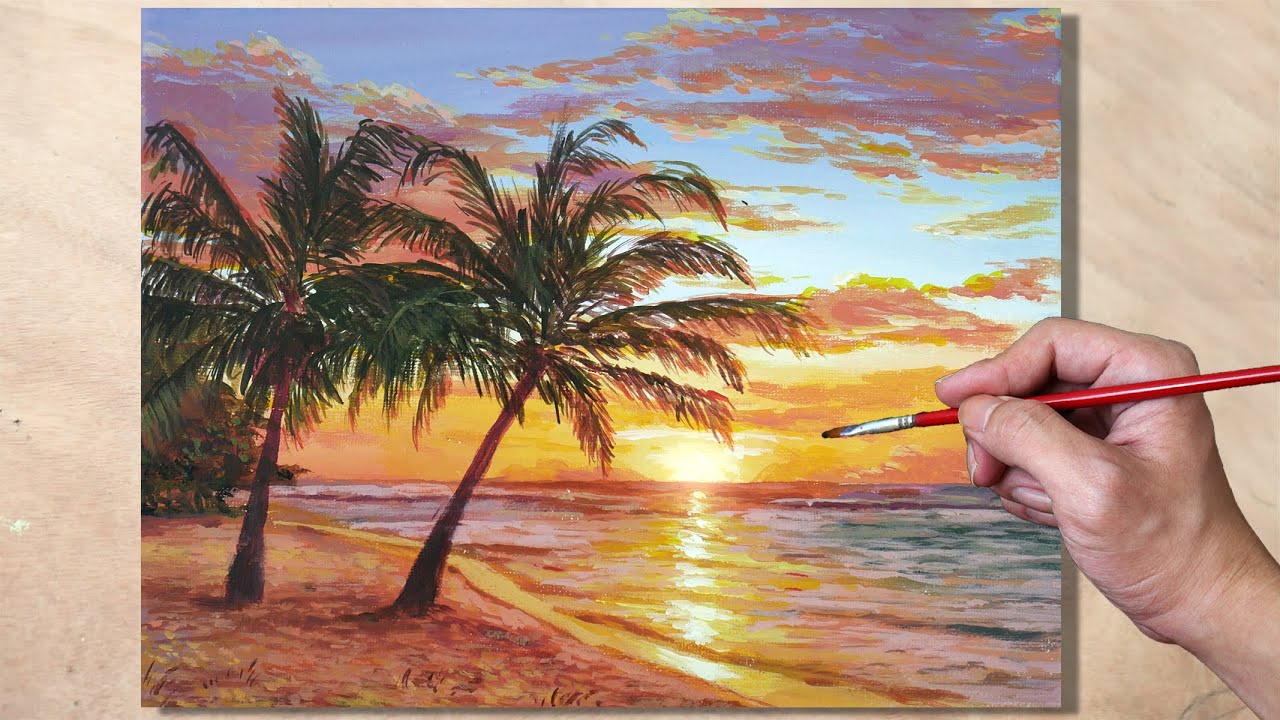This horizontal photograph captures an adult's light-colored right hand holding a red paintbrush with a metal tip and black bristles, poised in the foreground. The scene being painted is a serene beach at sunset, set against a light beige background that could be a wall or an easel. The beach scene features a vibrant, setting sun low on the horizon, casting a luminous yellow glow. The sky transitions from yellows and oranges near the sun to pinks and purples among the clouds, with the deeper sky fading into darker blue hues. The ocean reflects these colors in its wavy surface as it meets the sandy shoreline. The beach is adorned with two prominent palm trees: one leans out over the water, while the other stands closer inland, accompanied by visible footprints in the sand. The entire image conveys a peaceful, serene atmosphere with its harmonious blend of colors and natural elements.